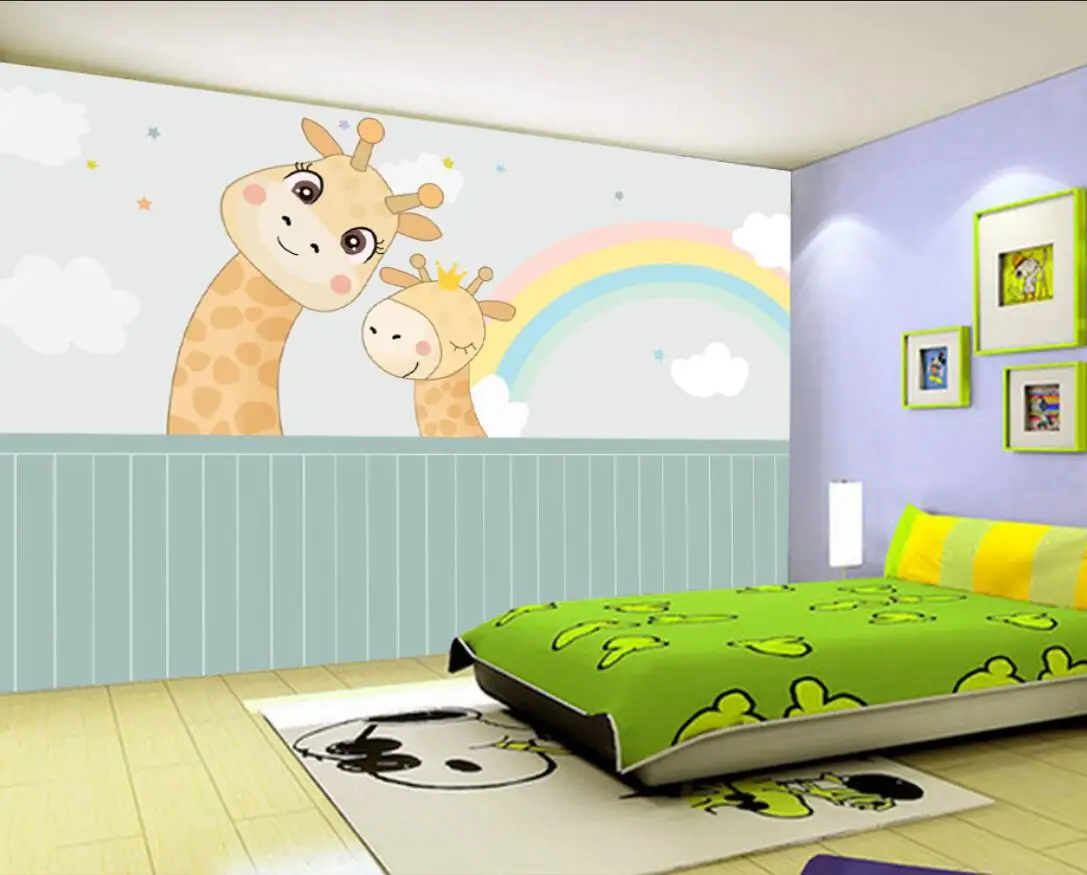The image depicts a children's bedroom, possibly AI-generated. The room features a half-paneled wall in light blue wainscoting with a vibrant mural above it, illustrating a smiling mama giraffe and a baby giraffe adorned with a gold crown. The mural also includes a colorful rainbow, fluffy clouds, and stars against a periwinkle blue backdrop. The bed is positioned against this wall and another wall painted in a similar blue shade. The bedding is lime green with lighter green designs, complemented by a large pillow with wide tan and yellow stripes. Above the bed on the adjacent wall, three framed artworks with distinct lime green borders display Snoopy, Mickey Mouse, and an unidentified character. Below, a Snoopy-themed rug partially extends under the bed, set on a light-colored wooden floor. The room also contains a blue lamp near the wall featuring the giraffes.